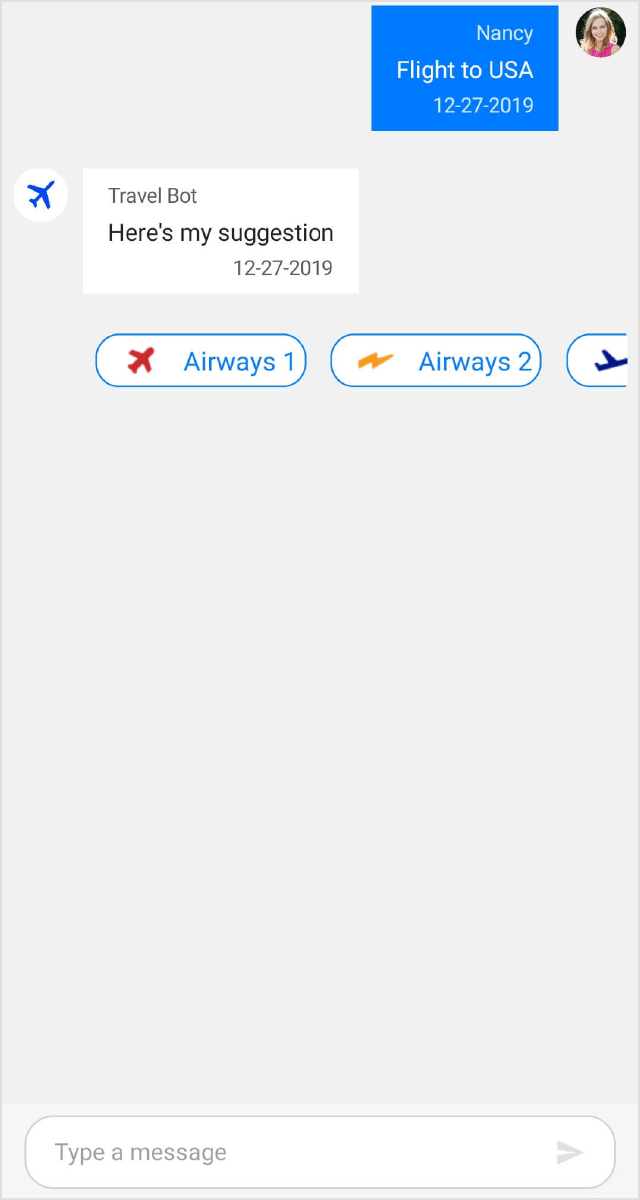This image is a screenshot featuring a predominantly white background. In the upper right corner, there's a portrait view of a woman with blonde hair wearing a pink shirt. To the left of her image, text reads "Nancy flight to USA 12-27-2019." Below this text is a white box that stands out against the gray background. Inside the box, there is an image of a blue airplane on the left side, and to the right in bold text it reads "Travel bought: here's my suggestion 12-27-2019."

Further down, there are two buttons. The first button is white with a blue outline border and blue text that reads "Airways 1," accompanied by a red airplane icon to the left. The second button is also white with a blue border and blue text that reads "Airways 2," featuring a yellow lightning bolt icon to the left.

At the very bottom of the screenshot, there is a text input box outlined in a thin gray line. Inside the box, light gray text prompts the user with "type a message," and an arrow points to the right.